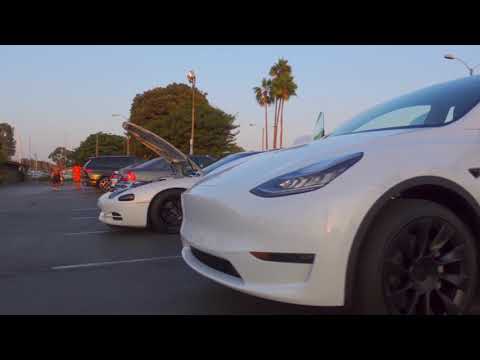This detailed image depicts a parking lot with a dark black pavement marked by white lines. The photograph is taken from a side view, showcasing a lineup of cars. In the foreground to the right, there is a compact white sedan with one wheel visible. Directly behind it, there's another white car with its hood open, suggesting maintenance or a mechanical issue. Further down the line is a gray vehicle, and additional cars can be seen fading into the distance, leading into the background.

The backdrop features a mix of very tall palm trees and broader, larger trees. The sky overhead is a gradient of clear blue, growing lighter near the horizon, indicating the approach of evening. The lighting is subdued, giving the picture a less bright appearance as the sun begins to set, casting a warmer tone across the scene.